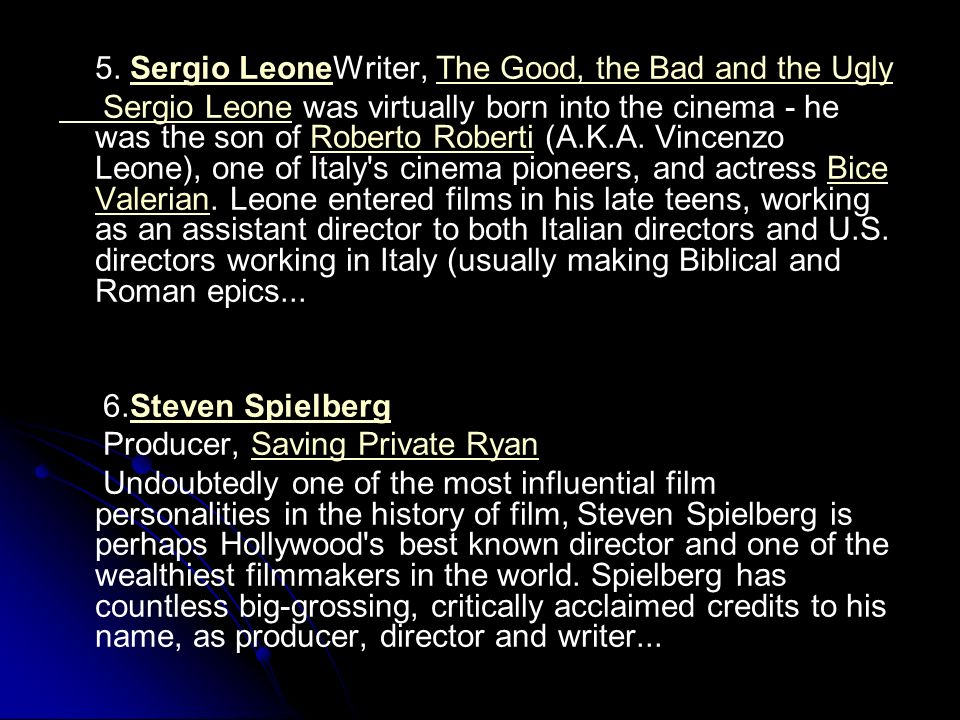The image resembles a slide from a presentation, featuring a predominantly black background with a striking, vibrant dark blue element in the bottom left corner that partially forms a circle with some rings. The slide is text-centric, with all words in a contrasting white typed font for clear readability. The text is organized into two distinct numbered paragraphs. 

The first paragraph, marked with the number 5, details Sergio Leone, a renowned writer. It prominently mentions "The Good, the Bad, and the Ugly" and provides a brief biography, emphasizing that Sergio Leone was virtually born into cinema. He was the son of Roberto Roberti (also known as Vincenzo Leone), one of Italy's cinema pioneers, and actress Bice Valerian. His early career involved working as an assistant director on both Italian films and American films shot in Italy, including many biblical and Roman epics.

The second paragraph, labeled with the number 6, focuses on Steven Spielberg in the role of producer, specifically highlighting his work on "Saving Private Ryan." It underscores Spielberg's significant influence in the film industry, labeling him as one of the most influential film personalities in history. Additionally, it notes his status as one of Hollywood's best-known directors and one of the wealthiest filmmakers. Spielberg's extensive career includes numerous high-grossing and critically acclaimed works in various capacities, including producer, director, and writer.

Overall, this slide offers a concise yet rich biographical insight into the careers and contributions of Sergio Leone and Steven Spielberg, set against a visually impactful black and blue background, designed for high contrast and readability.